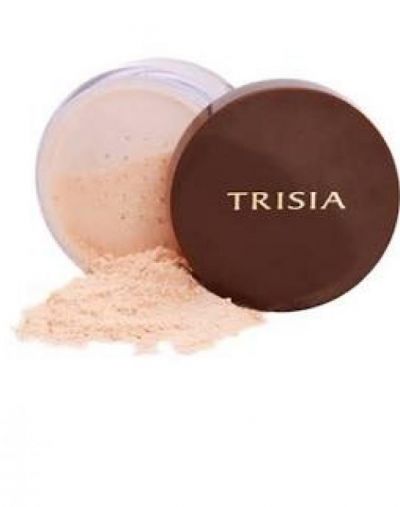In this detailed, edited photograph, we see an open cylindrical container of a light orange or peach-colored powder—a makeup product, potentially blush. The fine, ground powder spills out artistically onto the blank white table below from its horizontal position, resembling a small, intentional mound. The container's design includes a transparent base and a dark brown cap, which has rolled aside. The cap features the brand name "TRISIA" in light-colored font. The image conveys a sense of deliberate arrangement, emphasizing both the powder spilling out and the stylish, sleek design of the container.